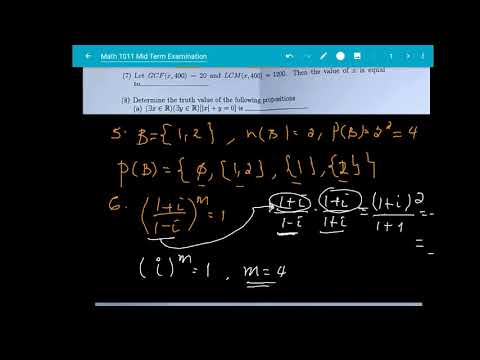The image depicts a virtual or hybrid educational medium with a solid black background, resembling either a computer screen or a chalkboard. Near the top of the square, landscape-oriented image, there is a blue horizontal strip featuring the text "Math 1011 Midterm Examination" prominently, along with several small, white navigation icons. Beneath this strip hangs a rectangular section of white paper with two math problems labeled "7" and "8," written in black text, indicative of an in-progress examination.

The blackboard or screen itself displays mathematical equations in two distinct sections. The upper equations are rendered in a light brown or gold color, while the lower equations, numbered "5" and "6," are written in a combination of white and light brown (or orange) chalk or text. The white, horizontal line separates the upper exam problems from the lower section, adding to the structured presentation of the material. The image has a photographic quality, capturing the clear details and organized layout of the displayed content.